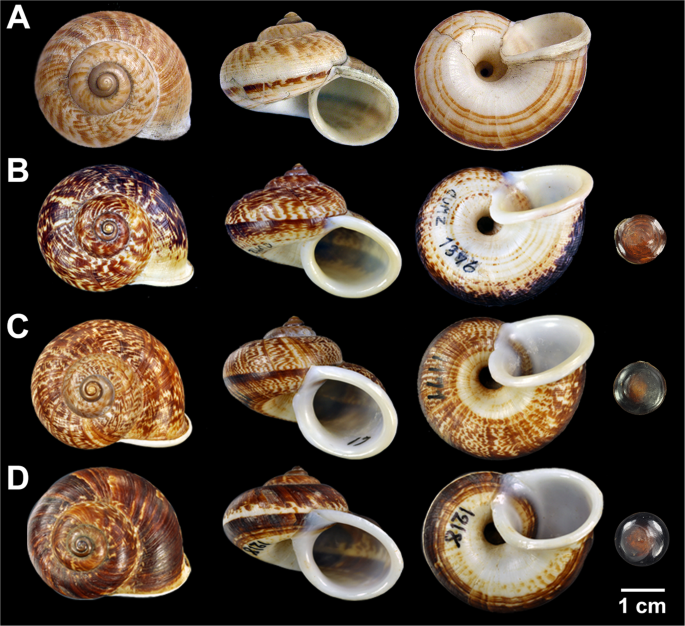A collage of twelve mollusk-like seashells, arranged in a 4x3 grid on a black background, labeled with white capital letters A through D from top to bottom. Each row displays three different views of four individual shells: the first column shows a side view of each shell, the middle column presents the underside with the entrance to the shell, and the last column offers another side view from a different angle, featuring the upper spiraled tip. Beneath these columns on the right, there are three small circles serving as a scale, marked with "1 cm" to highlight the petite size of the specimens. The shells themselves are similar in size but differ in color and pattern, exhibiting a range of browns, whites, and occasional hints of red and blue. The backgrounds and detail scales emphasize the natural diversity and intricate markings of each shell against a uniform dark setting.